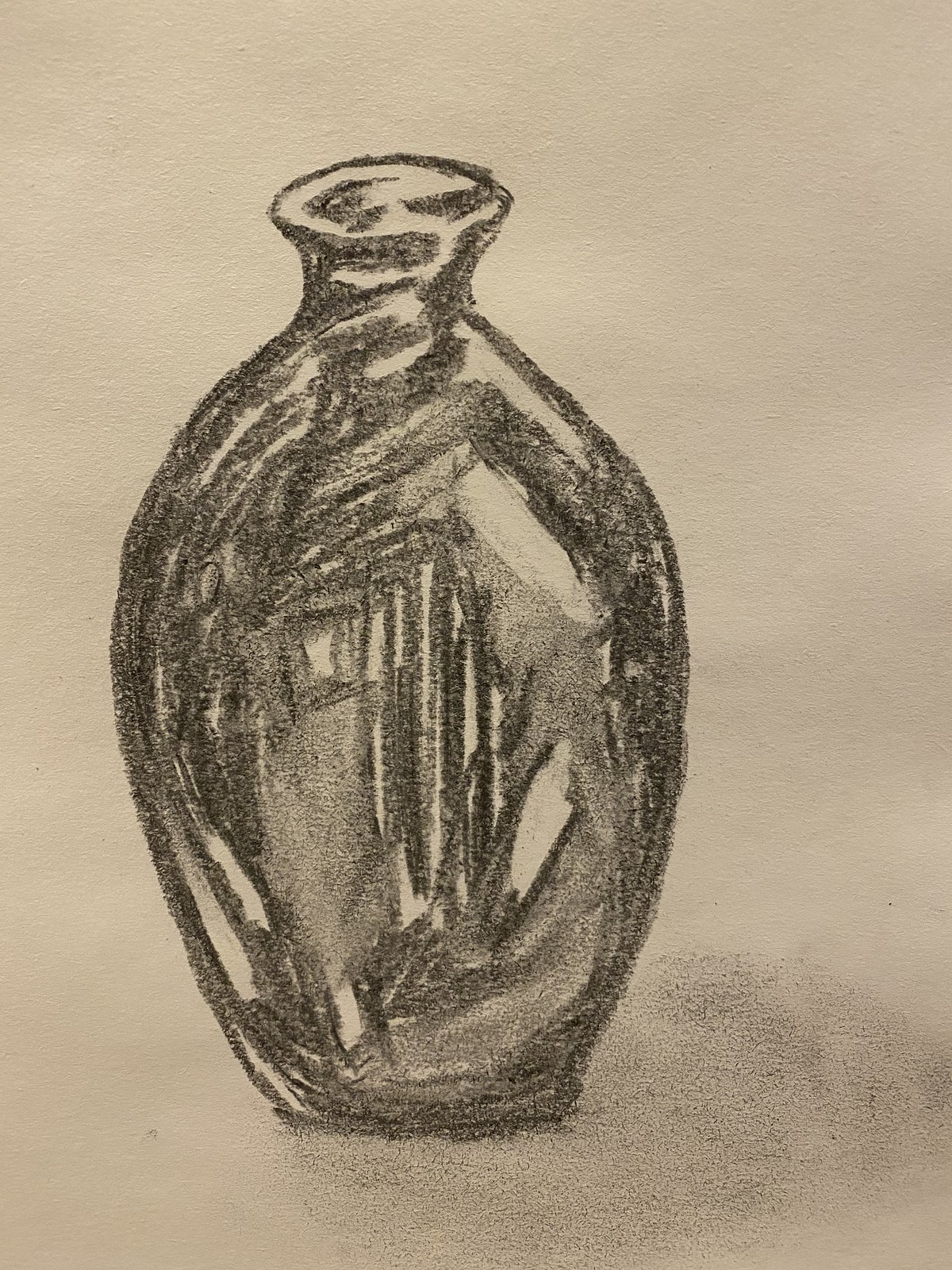This illustration features a black pot rendered with either pencil or charcoal. The artwork, in monochrome tones of black, white, and gray, depicts a pot with a broad, wide body, a small neck, and a narrow opening at the top. The base of the pot is relatively small, creating a distinct contrast with its wider midsection. The surface of the pot is adorned with jagged charcoal lines, adding texture to its appearance. Additionally, parts of the pot, particularly near the bottom right, exhibit rubbed-out areas, contributing to a sense of depth and character. The pot’s shadow on the ground shares this rubbed-out texture, blending into the off-white background of the surrounding paper.